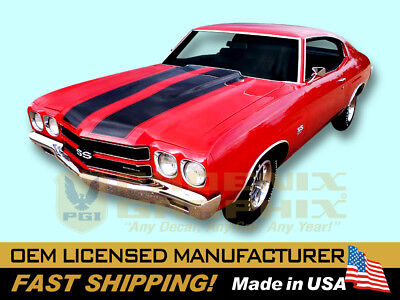The image is an advertisement featuring a glossy, red Chevrolet Malibu muscle car, reminiscent of the early 1970s. The two-door car boasts two thick black racing stripes running down the length of its hood, which includes a raised hood scoop in the center. The front end of the vehicle features a prominent chrome bumper and a black grille, accentuated by red paint between the grille sections. Two large, glass-lens headlights with chrome rings adorn each side of the front. The car is marked with "SS" emblems in chrome on the grille and sides, standing for Super Sport. The ad has a light blue background with some indistinguishable lettering and an emblem partially obscured by the car. Along the bottom of the image is a yellow and black banner stating, "OEM licensed manufacturer, fast shipping, made in the USA," accompanied by a small American flag.